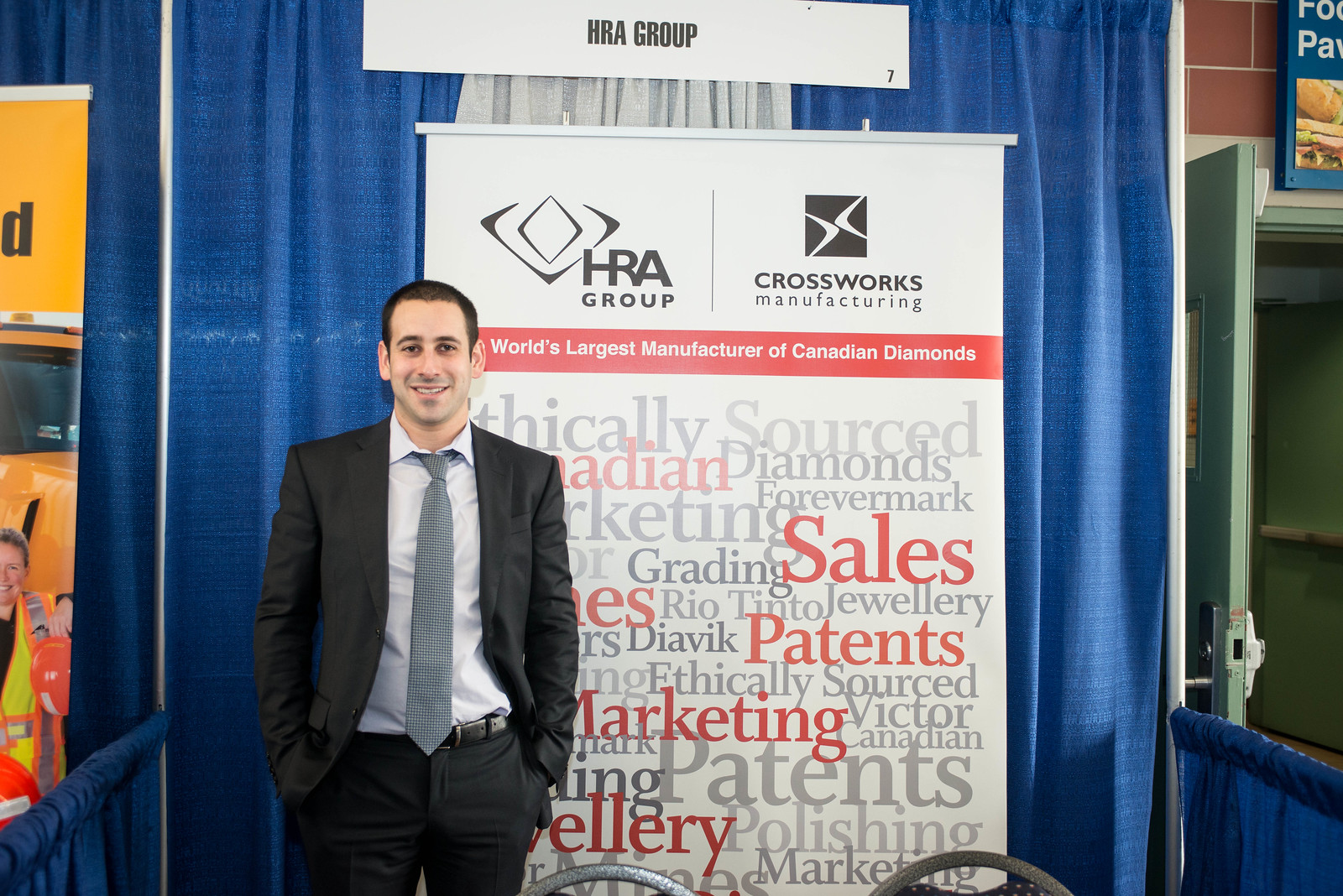The photograph depicts a man with short, dark hair, and very fair skin, standing and smiling in front of a large, freestanding white banner with a blue curtain backdrop, suggesting an indoor setting, likely a convention hall or conference booth. The banner, which is taller than the man, prominently displays the words "HRA Group" at the top, accompanied by a red band with a diamond shape and the text "Crossworks Manufacturing" underneath. It also features the slogan "World's largest manufacturer of Canadian diamonds" in prominent red letters. Below this, a cloud of various terms such as "ethically sourced Canadian diamonds," "Rio Tinto," "marketing," "sales," "patents," and "polishing" are scattered in different sizes and colors. The man is dressed in a dark gray suit, a light gray-blue shirt, and a gray patterned tie, with his hands in his pockets. On the left side of the image, another booth banner and the tops of metal-framed chairs are visible, while on the right, there's an open doorway. The overall ambiance is that of a professional convention or trade show with individual booths set up.